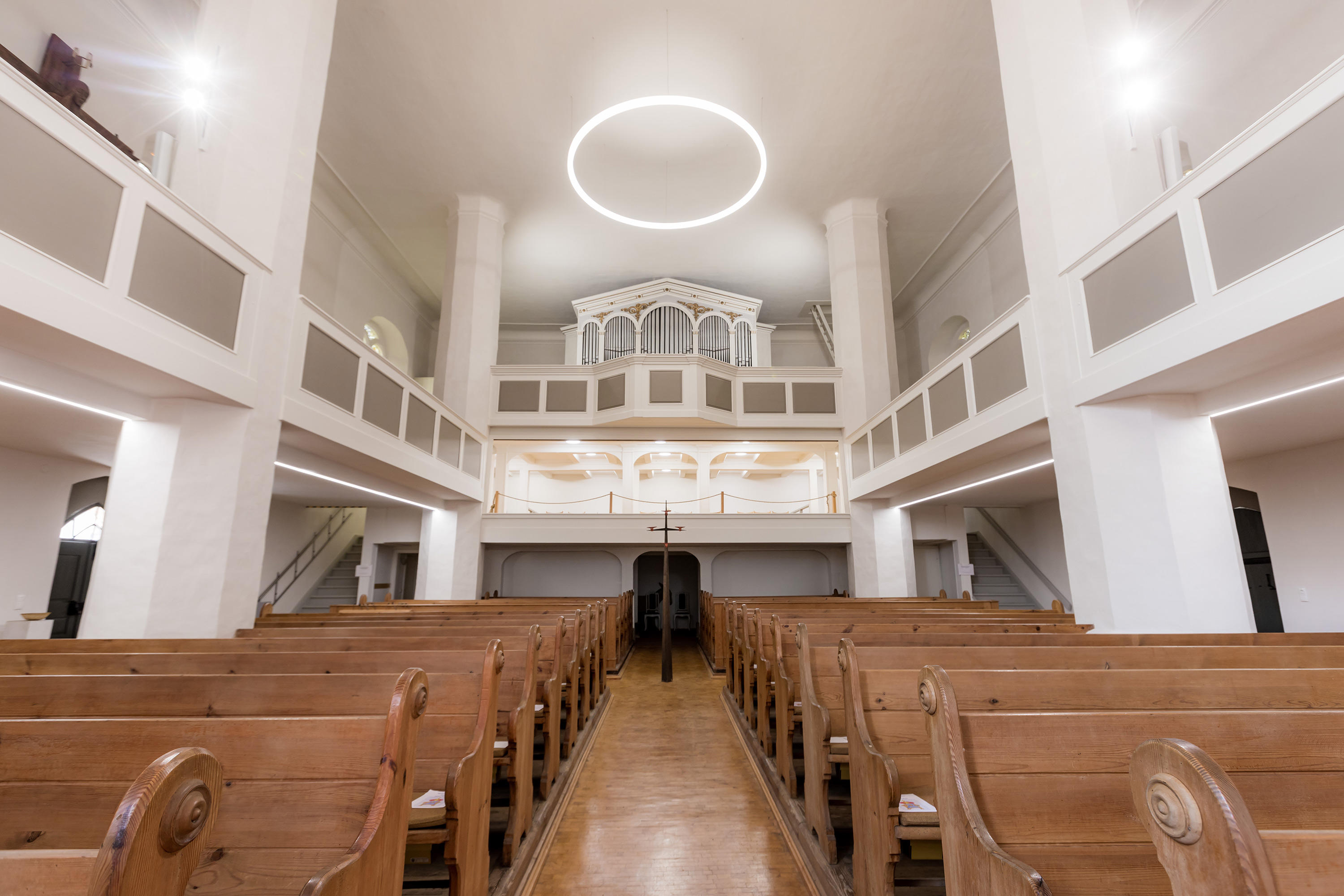This detailed color photograph captures the serene interior of a well-lit Christian church, taken from the pulpit looking towards the back. The symmetrical composition showcases rows of brown wooden pews lining both sides of the central aisle, which appears to be made of wooden flooring. In the distant background, a tall, thin wooden crucifix stands prominently. The church spans two stories, featuring white-painted upper levels supported by elegant white columns with gray square fronts. These upper balconies, likely intended for the choir, house pipes and are accentuated by a halo of light from white arches and a cornice above. The space is illuminated naturally through windows, casting soft light on the predominantly brown, white, and gray interior. The scene is devoid of people and text, focusing purely on the architectural beauty and tranquil atmosphere of the sacred space.